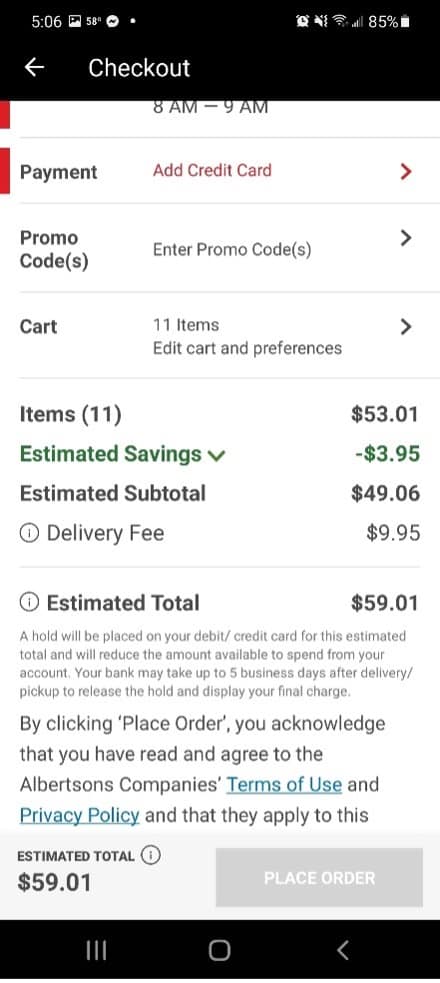This image captures the checkout page of an online shopping platform. At the top left corner, the page is distinctly labeled "Checkout." The main section of this snapshot showcases several essential features for completing a purchase. 

Prominently, there is a field for inputting a promo code to potentially reduce the overall cost. Below that, there is an area designated for entering credit card information to process the payment.

The snapshot indicates that a total of 11 items are in the cart. The detailed breakdown of costs reveals a subtotal of $53.01, with an estimated savings of $3.95, leading to a revised subtotal of $49.06. Additionally, a delivery fee of $9.95 is applied, resulting in a final estimated total of $59.01.

Beneath these financial details, a note informs customers that a hold will be placed on their debit or credit card for the estimated total, reducing the available balance in their account. It mentions that the bank may take up to 5 business days after delivery to release the hold and finalize the charge.

At the very bottom of the checkout page, the estimated total of $59.01 is reiterated in the bottom left corner. Meanwhile, in the bottom right corner, there is a prominent gray rectangular button with the text "Place Order" centered within it.

Overall, the image effectively illustrates the crucial steps and financial summary involved in finalizing an online purchase.